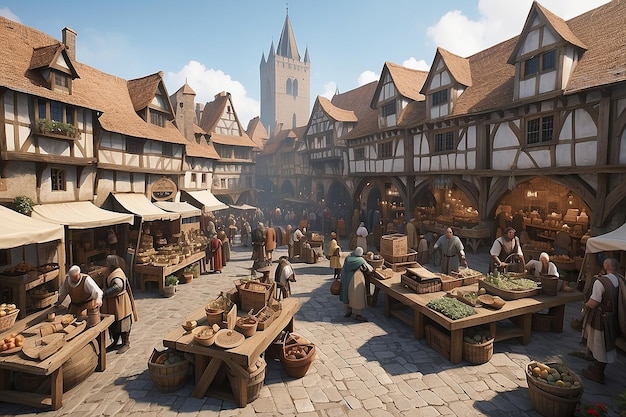The horizontally aligned rectangular image depicts a detailed scene from a realistic medieval-style video game. It features an outdoor market set within an old village, where men dressed in brown and white gowns are working and selling goods. These villagers are set up along a stone-paved walkway flanked by rows of connected brown and tan buildings. The buildings, which have sloped triangular roofs and white-painted walls reinforced with dark wooden beams, extend upwards to create a picturesque scene of medieval architecture. 

On the left side of the image, tables under small canopies display various goods, while the right side has arched openings and wood stalls bustling with activity. Barrels filled with fruits are scattered around, and long wooden tables showcase items for sale, ranging from wooden buckets and lids to fresh produce and fish. 

Near the image's center, a taller building with a steeple, resembling a castle tower, stands prominently in the background, adding to the medieval ambiance. Shoppers weave through the market, examining the sellers' displays against the backdrop of clear blue sky adorned with a few white clouds peeking over the rooftops.